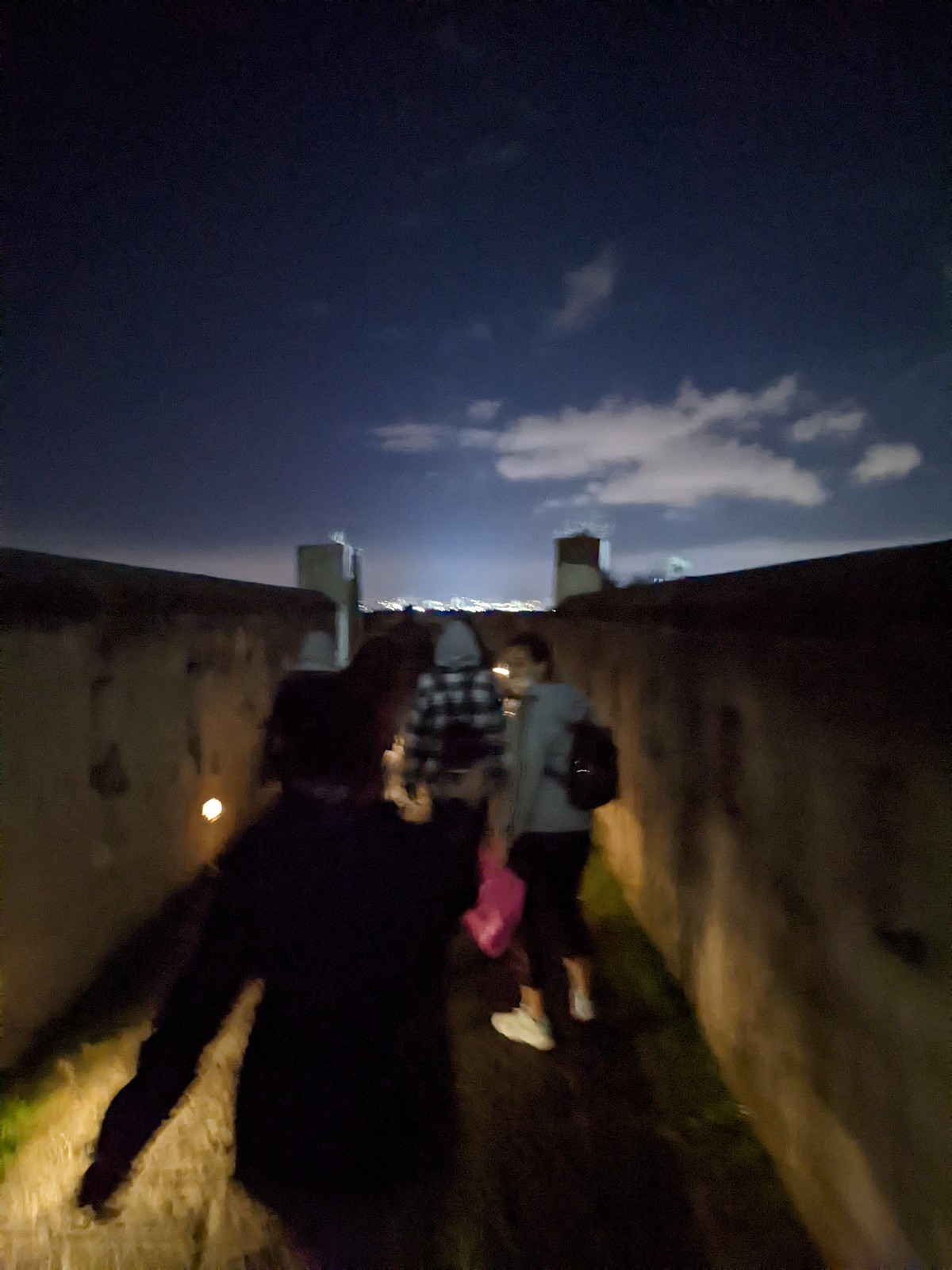In this somewhat blurry photograph, taken outdoors during the evening transitioning into nighttime, the deep blue sky is accentuated by patches of light gray clouds situated towards the center right. The image captures a group of young adults walking along a narrow bridge or possibly the parapet of a tower, characterized by its high walls that extend above their heads.

In the foreground, a person dressed in a black jacket is seen walking ahead. Just in front of them, a woman is visible, clad in a gray hooded jacket, black capri pants, white sneakers, and a black backpack. She is also carrying a distinct pink bag. Leading the group, another individual is wearing a hood and a plaid jacket, accompanied by a backpack, as they move forward along the elevated, enclosed pathway. The tall walls create a sense of separation from the surroundings, directing focus on the group navigating through the dimly lit passage.